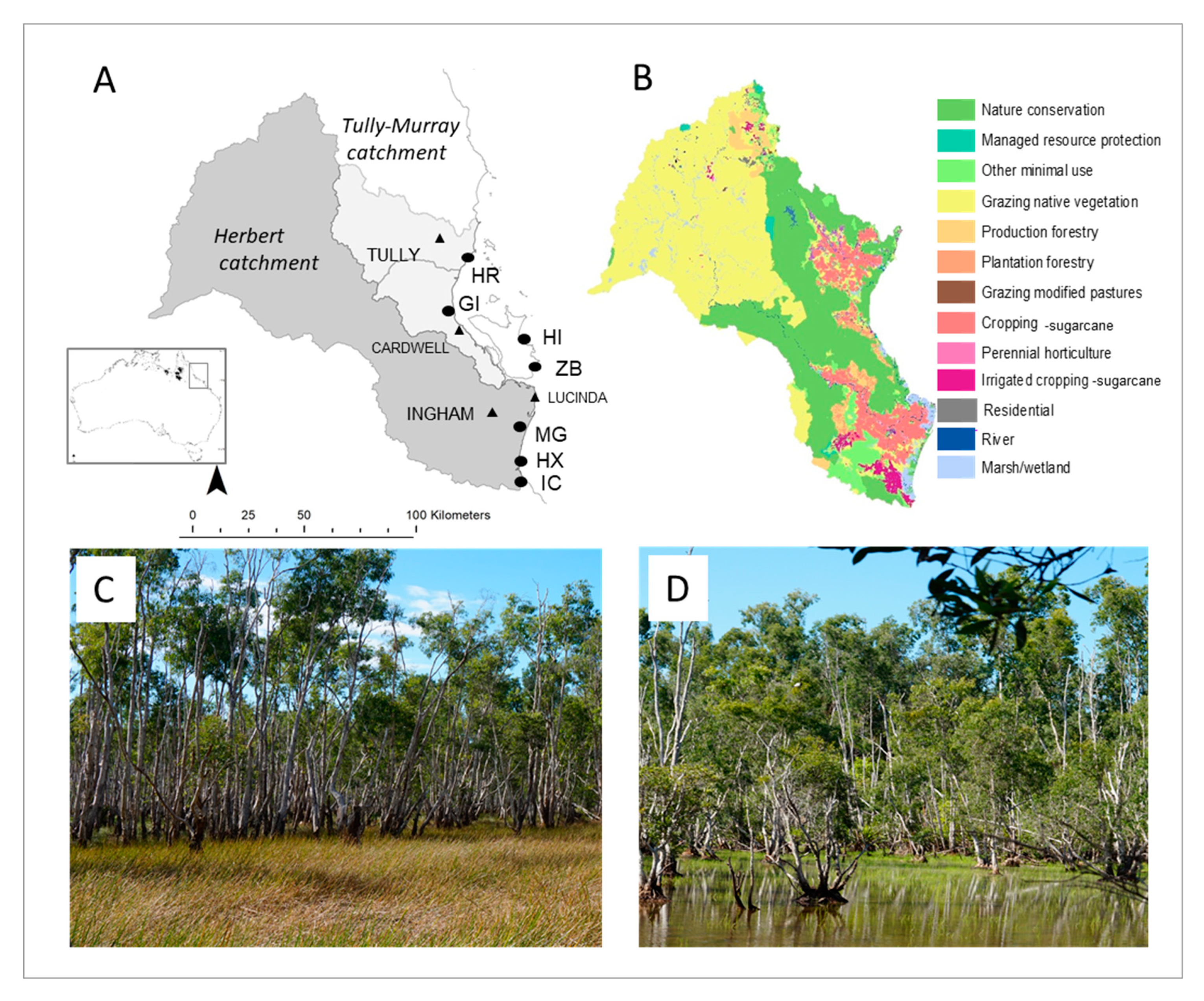The image is a detailed infographic likely from a geography textbook, divided into four distinctive sections labeled A, B, C, and D. 

- **Section A:** Features a black and white map highlighting various catchment areas such as Herbert Catchment, Tully-Murray Catchment, Tully, Cardwell, Agnum, and Cinda, along with some other marked locations.
  
- **Section B:** Presents the same geographical map as in Section A but utilizes a vibrant color-coding system to delineate different land uses. These categories include Nature Conservation, Managed Resource Protection, Other Minimal Use, Grazing Native Vegetation, Production Forestry, and Grazing Modified Vegetation, with a variety of colors representing each category. The map is accompanied by a color key on the right side.
  
- **Section C:** Displays a color photograph showing prairie grass in the foreground, a line of uniformly sized trees, with some slightly taller trees, all set against a backdrop of blue sky.
  
- **Section D:** Includes another color photograph that portrays a marsh area dominated by a small lake with trees growing out of the water and a forested area in the background.

This comprehensive layout visually communicates the different zones and land uses in a specific geographical area through detailed maps and corresponding landscape images.